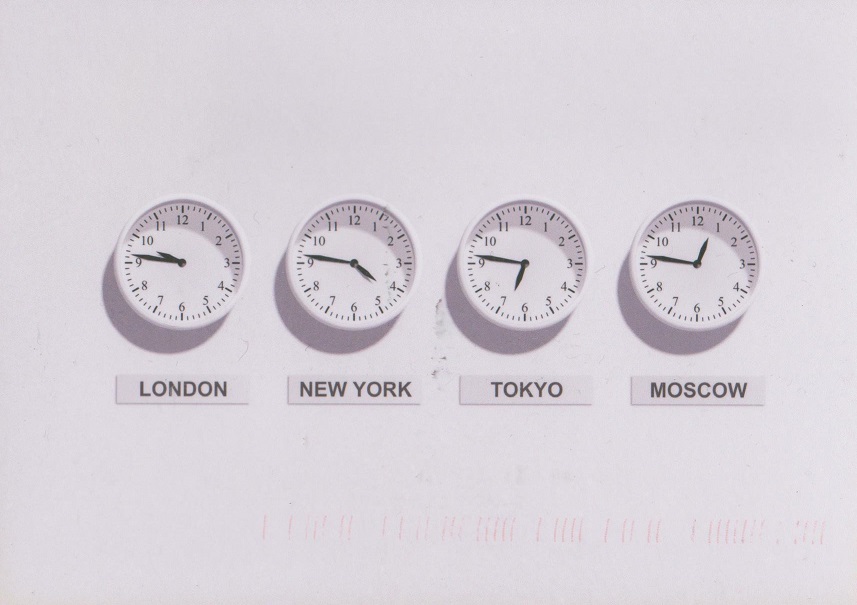The image is a photograph of four small, circular, analog clocks arranged in a row on a completely white wall. Each clock displays a different time and is labeled underneath in black font corresponding to major cities and their respective time zones. From left to right, the labels read London, New York, Tokyo, and Moscow. The clocks have white faces, black hands, and black numbers. The time displayed on each is as follows: London shows approximately 9:47, New York is at 4:47, Tokyo reads 6:47, and Moscow indicates 12:47. Crescent shadows appear below each clock, extending down and to the left. At the bottom of the image, red markings run horizontally across, adding a visual element to the scene that might suggest it is a postcard or a photographed print. The entire setup occupies about a third of the landscape-oriented picture.